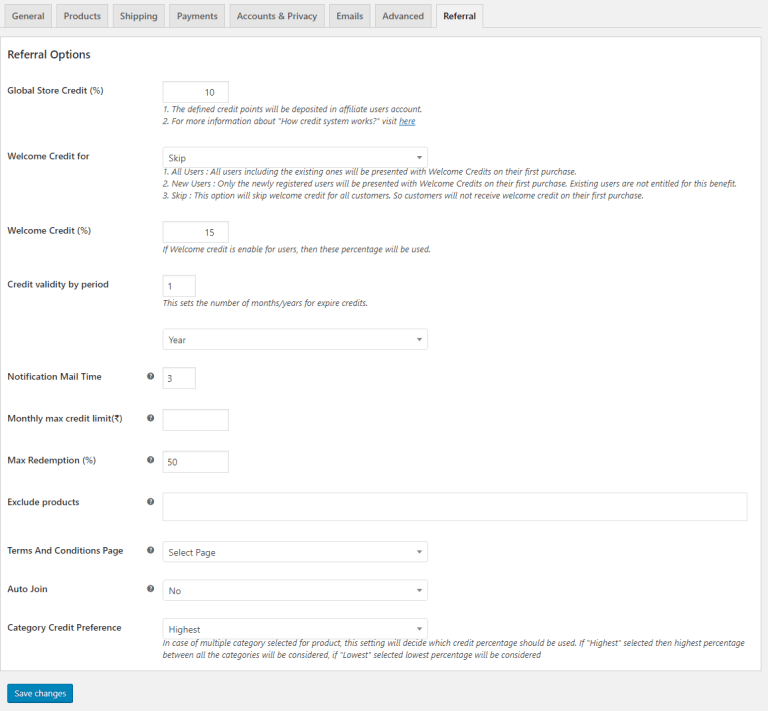This screenshot displays a webpage containing various settings for a particular website. At the top, there are multiple tabs for different sections, including General, Products, Shipping, Payments, Accounts and Privacy, Emails, Advance, and Referral. The Referral tab is currently selected, evidenced by its lighter color and bold, black font compared to the regular black of the other tabs.

The page is titled "Referral Options" on the left-hand side. Below the title, several adjustable settings are listed, such as:

- Global Store Credit: Contains a box for inputting the percentage, with an example value of "10".
- Welcome Credit Percentage
- Credit Validity by Period
- Notification Mail Time
- Monthly Max Credit Limit
- Max Redemption Percentage
- Exclude Products
- Terms and Conditions Page: Likely contains a link to the terms and conditions.
- Auto-Join
- Category Credit Preference

At the bottom of the list, a blue "Save Changes" button is visible, allowing users to save any modifications made.

Adjacent to each option, there are corresponding input boxes and additional information where necessary. For example, under "Global Store Credit Percentage," a box with the value "10" is provided, along with two explanatory notes: 
1. "The defined credit points will be deposited in affiliate user’s account."
2. "For more information about how the credit system works, visit here." The phrase "visit here" is a clickable hyperlink in blue, directing users to further details about the credit system.

The overall background of the webpage is primarily white, while the outer areas are highlighted in a whitish-green color.